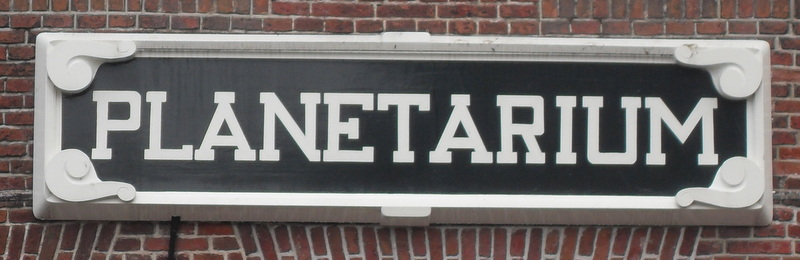The image depicts a sign affixed to a building constructed with reddish-brown bricks accentuated by light-colored masonry. The sign itself is framed with what appears to be a metallic border, featuring intricate white lines that resemble question marks in each of the four corners. Within the frame, a black plaque prominently displays the word "PLANETARIUM" in large, white capital letters. Extending from the bottom of the sign is a black cord suggesting it may be connected to a power source, possibly to illuminate the sign at night. The composition captures the blend of architectural textures and the simple yet attention-grabbing design of the planetarium sign.